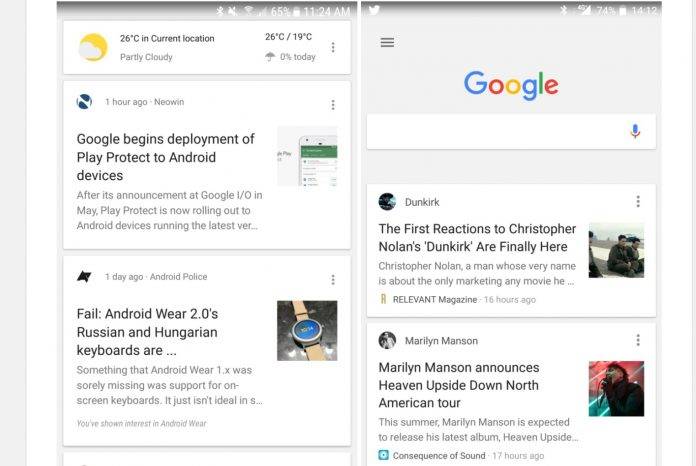In the given image, a detailed layout is presented within a box divided into two columns, bordered distinctly on both sides. The left border is defined by a prominent thick gray line extending from the top to the bottom, while the right border is subtly marked by a thin line.

### Left Column:
At the top, the current weather is displayed, indicating a temperature of 26 degrees Celsius with a partly cloudy condition. This is visually represented by an icon showing a sun partially obscured by a cloud. Beneath this, the temperature range for the day is provided, spanning from a high of 26 degrees Celsius to a low of 19 degrees Celsius, with a precipitation probability of 0%. Following this weather information, there is a section detailing recent updates:

- **One Hour Ago in Neowind**: An announcement that Google has begun the deployment of Play Protect to Android devices, initially disclosed during Google I.O. in May. The service is now rolling out to Android devices running the latest version, though the text is truncated and cuts off.

- **Another Box Below**: This section reports on the failings of Android Wear 2.0, particularly emphasizing the absence of Russian and Hungarian keyboard support, a feature that was notably missing in Android Wear 1.X.

### Right Column:
At the top of the right column, the word "Google" is prominently displayed, followed by a search field for conducting queries on Google. As you scroll down, there are two major headlines:

- **Dunkirk**: A brief description mentions that the first reactions to Christopher Nolan's film "Dunkirk" have been released.

- **Marilyn Manson**: An announcement about Marilyn Manson's upcoming North American tour, which is intriguingly titled "upside down."

This detailed caption captures all elements of the image, including visual features and text-based content, providing a comprehensive description.